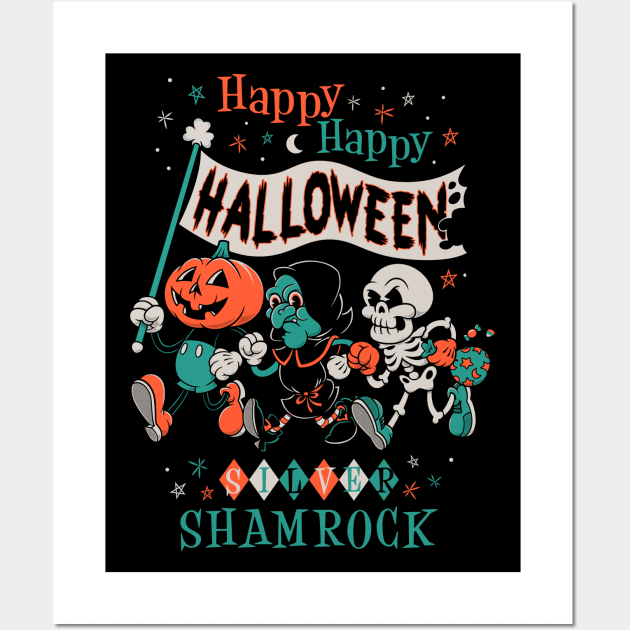This vibrant Halloween-themed poster features a black background with an array of colorful details. At the top, the word "Happy" is prominently displayed in orange, followed by another "Happy" in turquoise slightly offset to the right. Surrounding these words are whimsical white, turquoise, and orange stars, a crescent moon, and dotted accents. Below, a white banner adorned with black letters spells out "Halloween," attached to a turquoise pole topped with a three-leaf clover.

Centered on the poster, three animated characters hold hands while carrying the "Halloween" banner. From left to right, they include a pumpkin-headed figure dressed in turquoise shorts with two white buttons and large orange shoes; a witch-like character with a turquoise face, black puffy hat, black dress with orange trim, and turquoise-trimmed black shoes; and a skeleton character holding an orange-starred turquoise bag, wearing turquoise shoes. Beneath this lively trio is the phrase "Silver Shamrock," silver in a diamond-shaped pattern and shamrock in turquoise, accompanied by additional stars and dots for a festive touch.